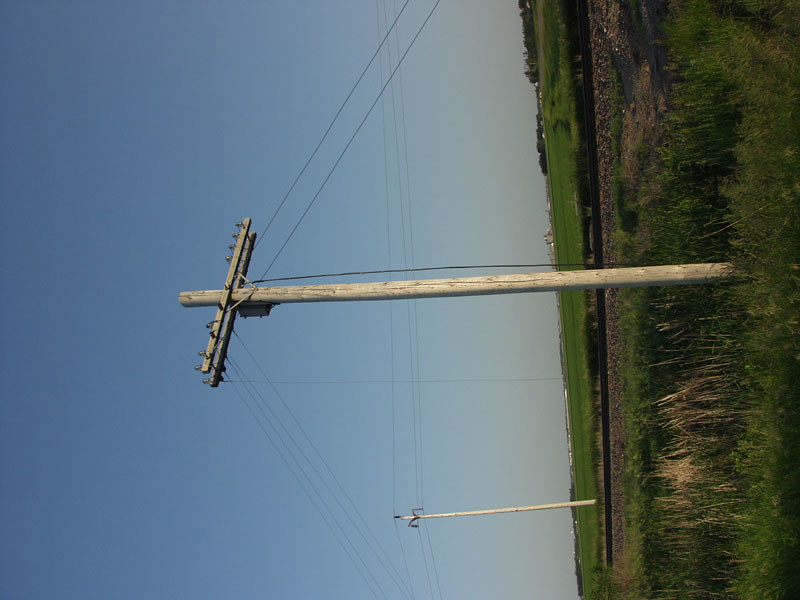The image, oriented sideways, depicts a scene from the outskirts of a city in a rural, open field. Dominating the foreground are two wooden posts, gray in color, that support an intricate network of black power lines arrayed in various directions. One post features a cylinder and multiple small, bell-like insulators arranged in pairs on both a front and back bar of wood, with power lines extending from these insulators—two lines in the front and four in the back. Right in front of the posts, the foreground reveals railroad or train tracks bordered on the left by dirt and rocks, and leading into a ditch filled with mostly green vegetation spotted with brown weeds. The expansive field, stretching out in the distance, features patches of both cut and overgrown grass as well as scattered areas of bare soil. Some distant buildings or city structures are faintly visible on the horizon. The sky above transitions from a light to dark blue, with indications that the sun may be setting, casting a serene yet expansive backdrop to the scene.